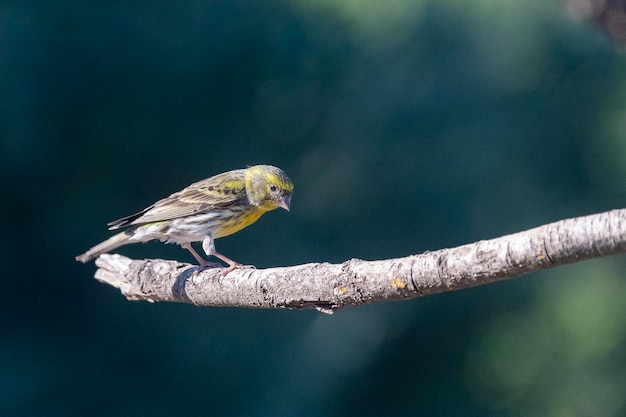In this detailed daytime outdoor photograph, a striking bird is the focal point as it perches on a prominent tree branch extending from the right side towards the left. The branch, which is devoid of leaves, displays a light brown hue and provides a solid perch for the bird, which is positioned near its end. The bird is depicted in a side view with its body facing left and its head turned slightly back, as though glancing over its shoulder. The bird's plumage features vivid yellow and gray tones, with a yellow belly, yellow markings around its eyes, and patches of yellow on its wings, contrasted by the primarily gray and white sections of its body. It also sports a small, beak and light pinkish-orange feet. Despite the blurred and somewhat dark blue-green background, which suggests a sky mottled with indistinct trees, the image clearly emphasizes the bird and branch, leaving the background in soft focus to highlight the detailed beauty of the scene.